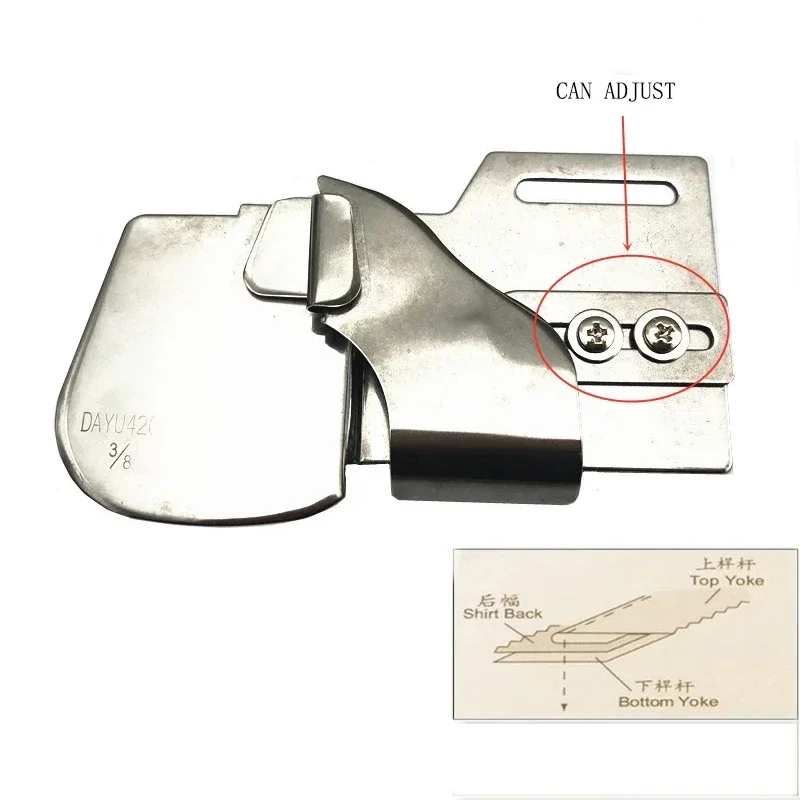The image features a predominantly white background, with a detailed mechanical component centered on it. The main object in the image is a shiny, silver metallic piece, which includes various parts: a clip, a sliding section, and two screws positioned next to each other within this sliding section. This slide mechanism is highlighted by a red circle and an arrow, pointing out that it "can adjust." Additionally, there is an instructional diagram at the bottom of the image, consisting of tan rectangular shapes labeled with both English and Asian text. These labels identify different parts such as "shirt back," "top yoke," and "bottom yoke." Overall, the image seems to serve as an instructional guide for adjusting a particular metallic component, with an emphasis on the screws' adjustment capability.